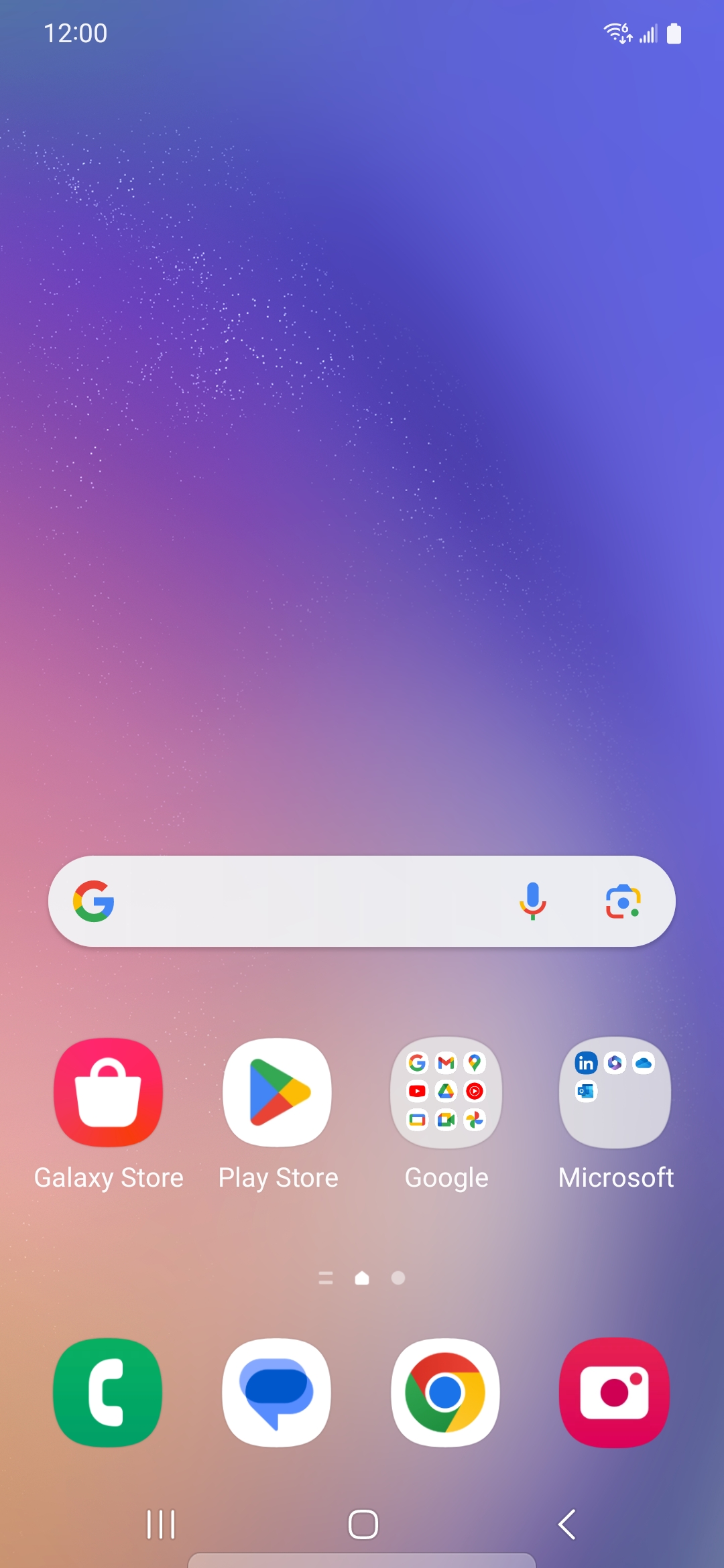This detailed caption describes a phone's homepage screenshot in vivid detail:

"This screenshot captures the homepage of a smartphone. In the top-left corner, the time reads 12:00 in white text. To the right, the status bar features a fully-charged battery icon, a Wi-Fi signal symbol, and a 4G or 5G service indicator.

The background showcases a gradient sunset theme, starting with a peach hue in the bottom left, transitioning to pink, then purple, and ultimately fading into blue at the top and top left corner.

At the lower center of the screen is a white Google search bar. On the left corner of the search bar is the Google logo, featuring the iconic 'G' in red, yellow, green, and blue colors. Adjacent to this logo are two icons: a microphone in rainbow colors, and a phone outline also in rainbow colors (blue, red, green, yellow).

Beneath the search bar are two rows of app icons. The first icon on the top left is a red box with a white shopping bag symbol, labeled 'Galaxy Store' in white. Next, there’s a white box with a play button symbol in red, blue, green, and yellow, labeled 'Play Store.'

Further down is a gray box displaying a grid of nine smaller icons, labeled 'Google' in white. Beside it is another gray box labeled 'Microsoft,' containing three icons in blue shades on the top row and one icon on the bottom row.

Further icons include a green box with a white phone symbol, a white box with a blue chat bubble, a white box featuring the blue Google logo (a circle with a blue center, a red top, green left side, and yellow right side), and a red box with a white camera icon."